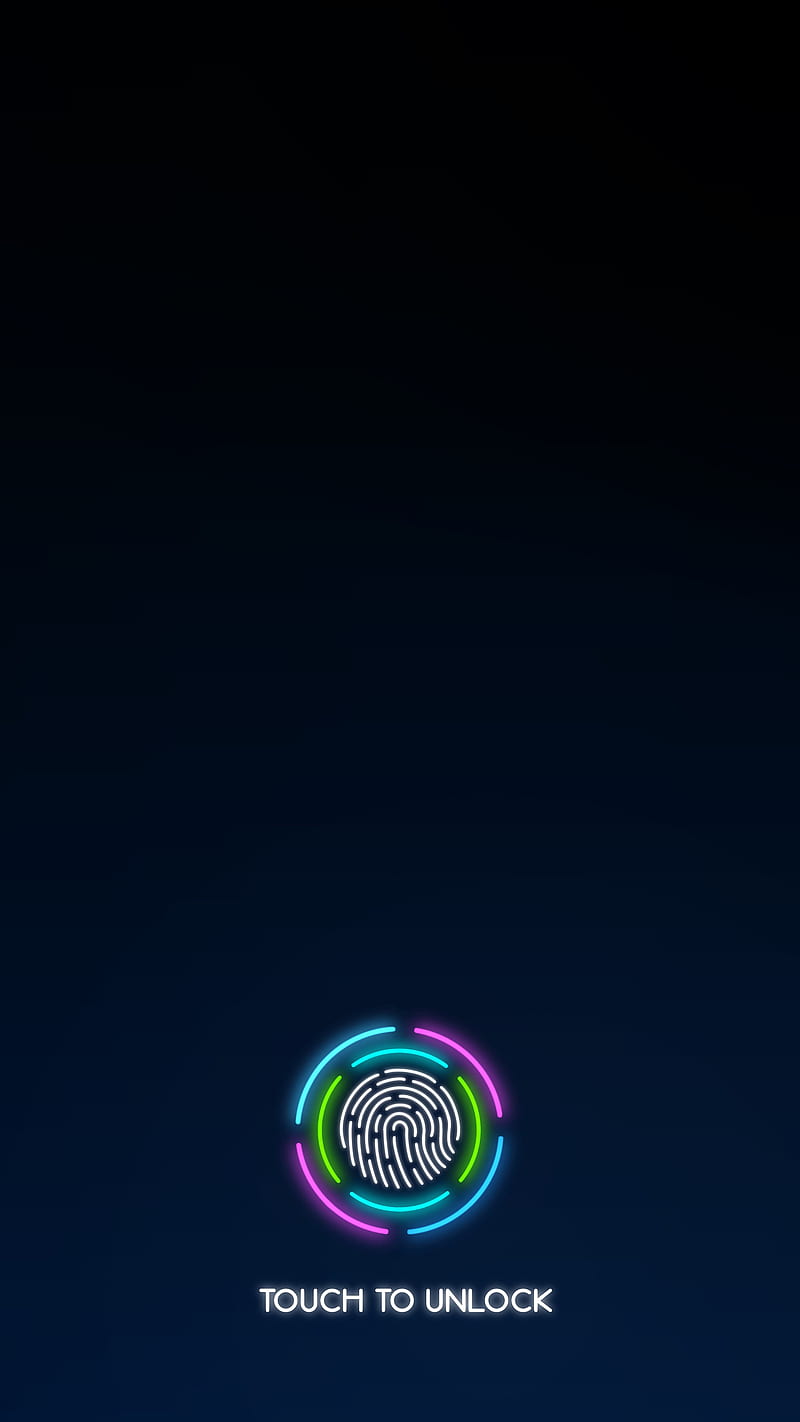This image, likely intended as a phone or media device lock screen wallpaper, features a sleek, modern design. The background transitions from a deep black at the top to a lighter blue gradient towards the bottom. Dominating the bottom quarter of the image is a prominently displayed, glowing fingerprint icon encircled by distinctive cyan, green, and magenta lines that form a complex pattern of concentric circles. These circles create an impression of dynamic motion and energy. Beneath the fingerprint icon, in all caps and a radiant white glow, are the words "TOUCH TO UNLOCK," emphasizing the function and interactivity of the screen. The overall aesthetic suggests a futuristic and technological theme, although the image lacks specific branding to indicate whether it's for an Android, Apple, or other device.